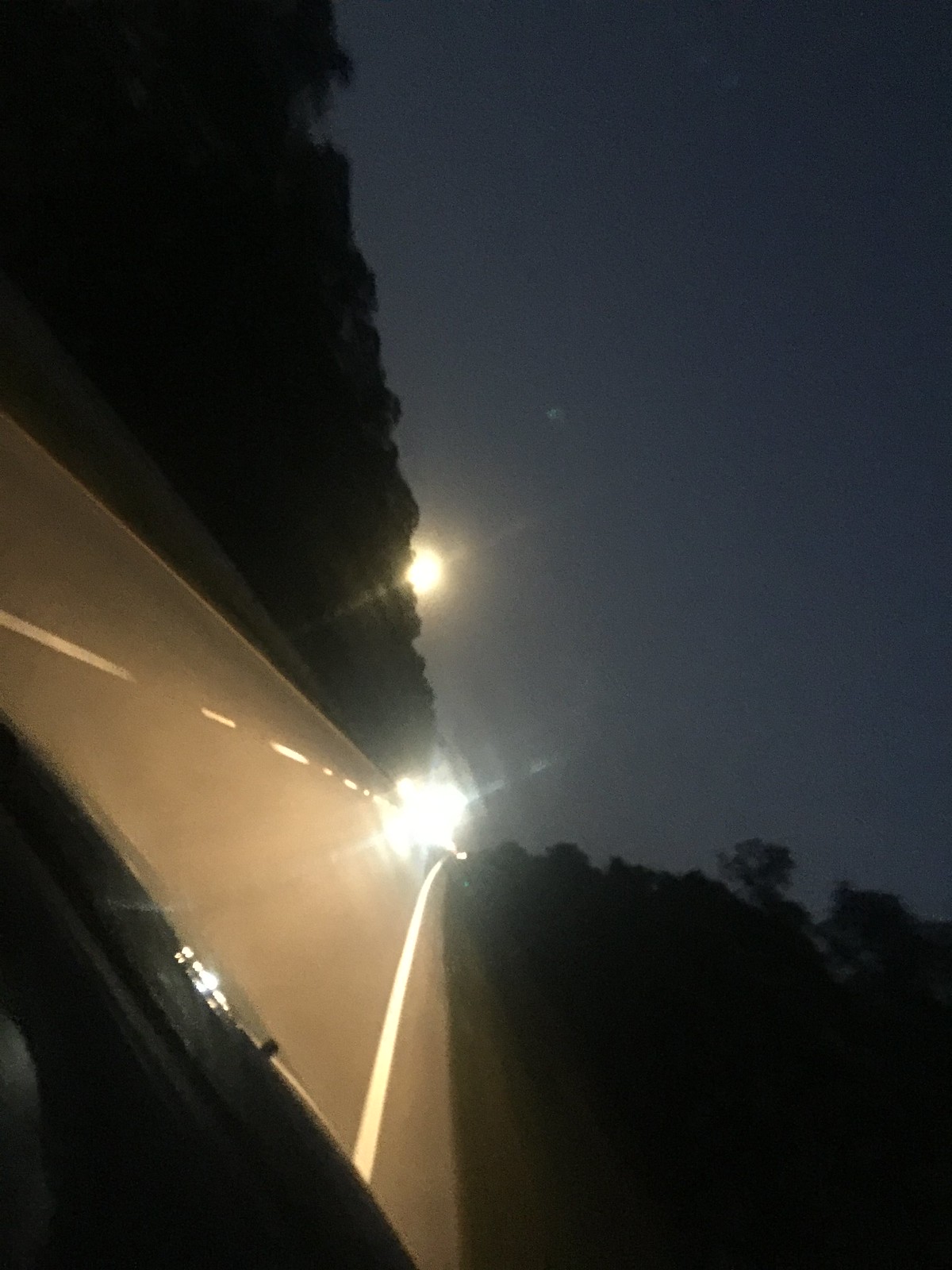A nighttime scene captured from the passenger seat of a moving car. The image is taken at a slight diagonal tilt, revealing the edge of the dashboard in the bottom left corner. The road ahead is faintly visible under the dim light, with headlights from several vehicles piercing through the darkness in the distance. A haze in the background that could be mistaken for the setting sun adds an enigmatic glow, but the overall scene remains dark. The surrounding landscape features dense grass and numerous trees lining both sides of the road. In the middle distance, a bright light source suggests an approaching vehicle, casting a surreal ambiance over the nocturnal drive.